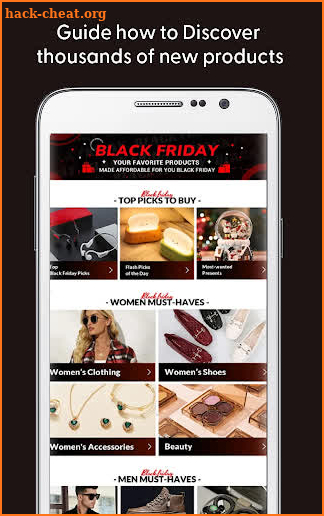The advertisement displayed is a vertical, mobile or online ad set against a black background with an orange border framing the entire image. In the top left corner, the text "hack-cheat.org" is prominently displayed in an orange font. Centrally aligned at the top in white font, it reads "A guide on how to discover thousands of new products."

Beneath this text, there is a photographic representation of a smartphone. The screen of the smartphone shows an advertisement for Black Friday. The ad headline reads "Black Friday" in bold red font on a black background. Below this, accompanying text states, "Your favorite products made affordable for you Black Friday." The screen is filled with various product images and categories.

At the top of the smartphone screen is the heading "Top picks to buy," showing three side-by-side images. The first picture showcases electronics, the second appears to feature toast or another ambiguous item, and the third is unclear.

Following this, there is a section titled "Women Must-Haves," highlighted with red italic writing above it (potentially reading "Black Friday"). This section includes four labeled photos arranged in a grid, with two across the top and two beneath. The categories within this section are:

1. Women's Clothing: Featuring a photo of a blonde woman wearing sunglasses and a plaid outfit.
2. Women's Shoes: Displaying a single style of slip-on loafer available in red, navy, and white colors.
3. Women's Accessories: Showcasing a full parure set of jewelry including ring, necklace, earrings, and bracelet.
4. Beauty: Highlighting a close-up image of makeup products.

Towards the bottom of the screen, partially cropped off, is the section "Men Must-Haves," revealing three categories; however, the labels for these categories are not fully visible.